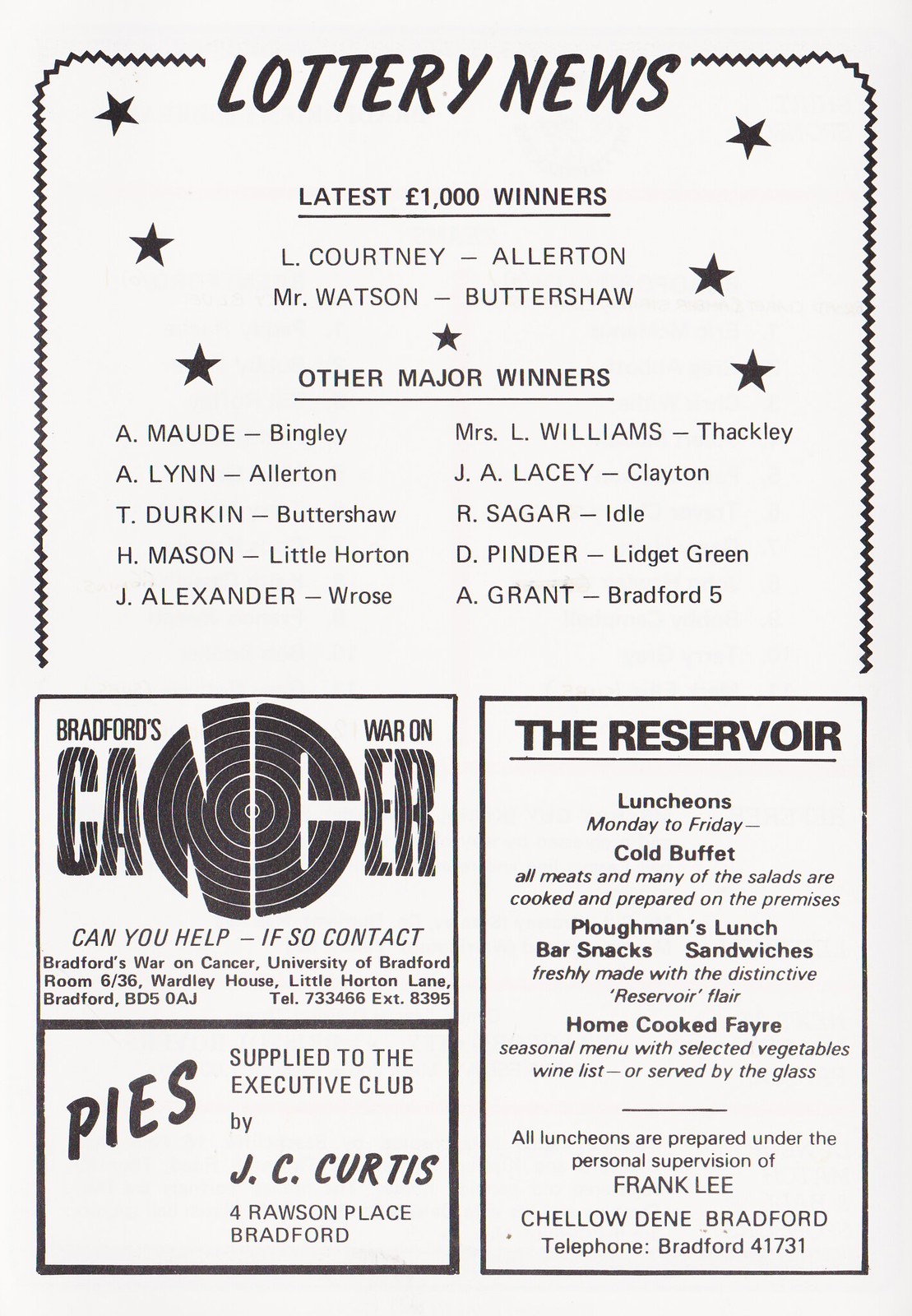This tall, rectangular flyer with an off-white background appears to be an announcement and advertisement page, possibly from a newspaper or magazine. At the top, bold, capital letters read "LOTTERY NEWS," accented by a zigzag border extending down both sides. Directly below, it announces the "Latest 1,000 Euro Winners: Elle Courtney Allerton and Mr. Watson Buttershaw," with small black stars adorning the sides. Beneath this, it lists "Other Major Winners," followed by the names of additional winners arranged in two columns of five names each.

On the lower portion of the flyer, to the left, there are two stacked advertisements. The top ad features a black record and reads "Bradford's War on Cancer," encouraging support and contact for the initiative. The second ad below it states, "Pies Supplied to the Executive Club by J.C. Curtis."

To the right of these ads, there is a larger, detailed advertisement for "The Reservoir," outlined by a black rectangle. Highlighted in bold letters, it promotes their lunch offerings from Monday to Friday, including a cold buffet with meats and salads prepared on-site. Additional details describe a "Plowman's Lunch," bar snacks, freshly made sandwiches, home-cooked fare, a seasonal menu with selected vegetables, and a wine list served by the glass. The ad emphasizes that all luncheons are prepared under the personal supervision of Frank Lee. Each section of the flyer is meticulously detailed and crafted to convey key information to the reader.